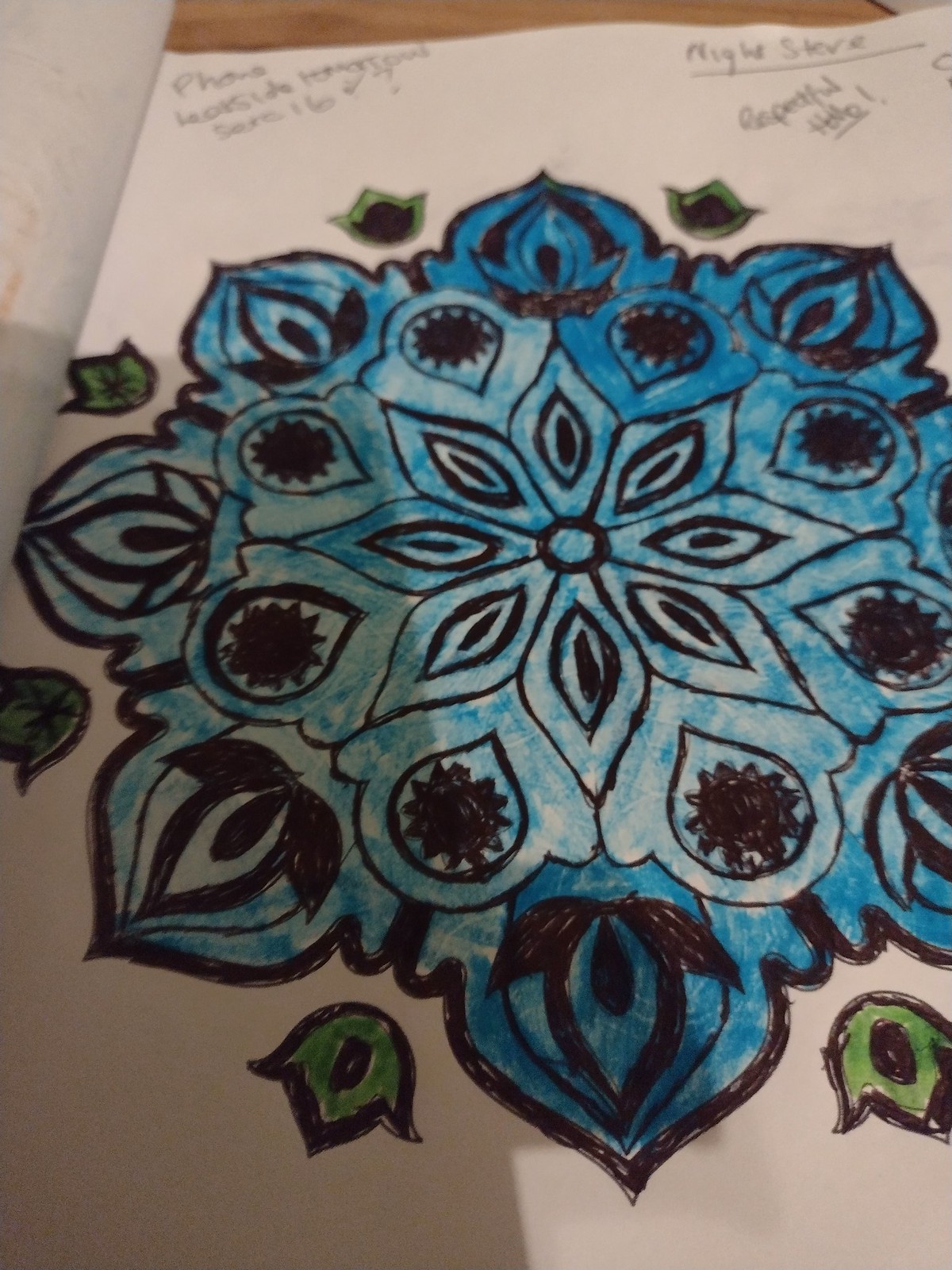This detailed illustration features various textual elements and floral imagery. In the top left corner, there is some text, while additional neatly arranged text is present in the top right corner. At the center of the image, a flower with multiple intricate petals is depicted. These central petals contain black markings, resembling hollow leaves with black dots at their centers. Surrounding these are additional petals with plaques at their tips, contributing to an elaborate design. The overall form resembles a lotus flower at its core. In the bottom left corner, there is a depiction of a bulb-like flower, characterized by its green interior.